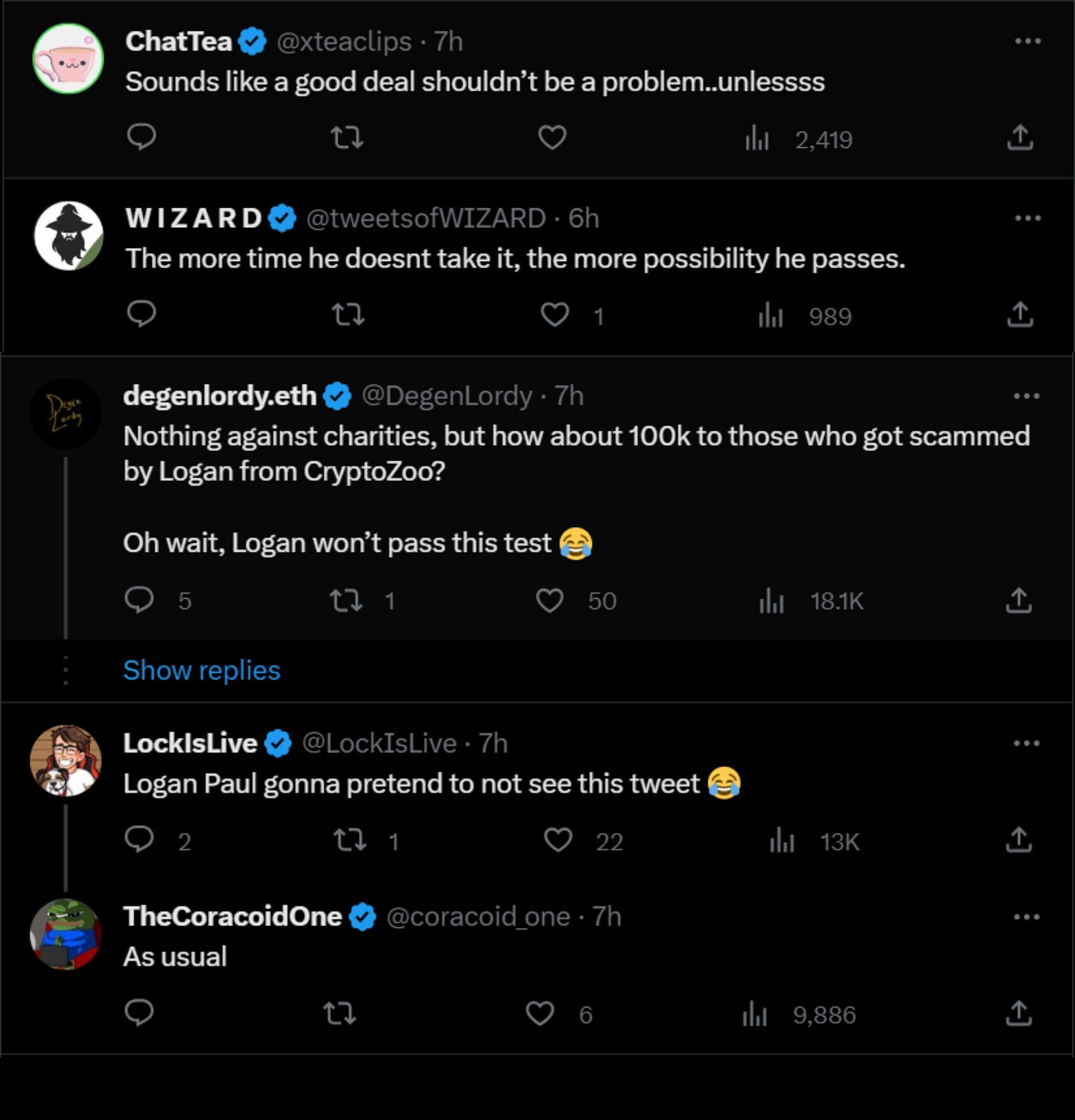**Caption Cleanup:**

---
At the top of the image, there is a pink teacup inside a white circle. Next to it, in white lettering, is the handle "@XTClips" with a blue checkmark, indicating a verified account. Beside this, it says "7 hours" ago in grey font. Below that, the text reads: 
"Sounds like a good idea, should be a problem... unlessssss."

Underneath, there is a depiction of a wizard wearing a black hat and sporting a black beard, reminiscent of the Wicked Witch from The Wizard of Oz. Next to the wizard, accompanied by a blue checkmark, it says: 
"The more time he doesn't take it, the more possibility he passes."

Further down, the username "@DEGENALORITY.eth" with a blue checkmark appears. The text under this handle reads: 
"Nothing against charities but how about 100k to those who got scammed by Logan from CryptoZoo? Oh wait, Logan won't pass this test 😂."

Beneath that, the phrase "luck is live" is displayed along with a cartoon image of a man with his dog. The tweet mentions:
"Logan Paul, gonna pretend to not see this tweet 😂."

At the bottom, the handle "@CORACOID_1" with a blue checkmark is visible. The accompanying text reads: 
"As usual."

Next to this, there is an image of a frog wearing a blue shirt.
---

This cleaned-up caption should offer a clear and detailed description of the original image and text content.